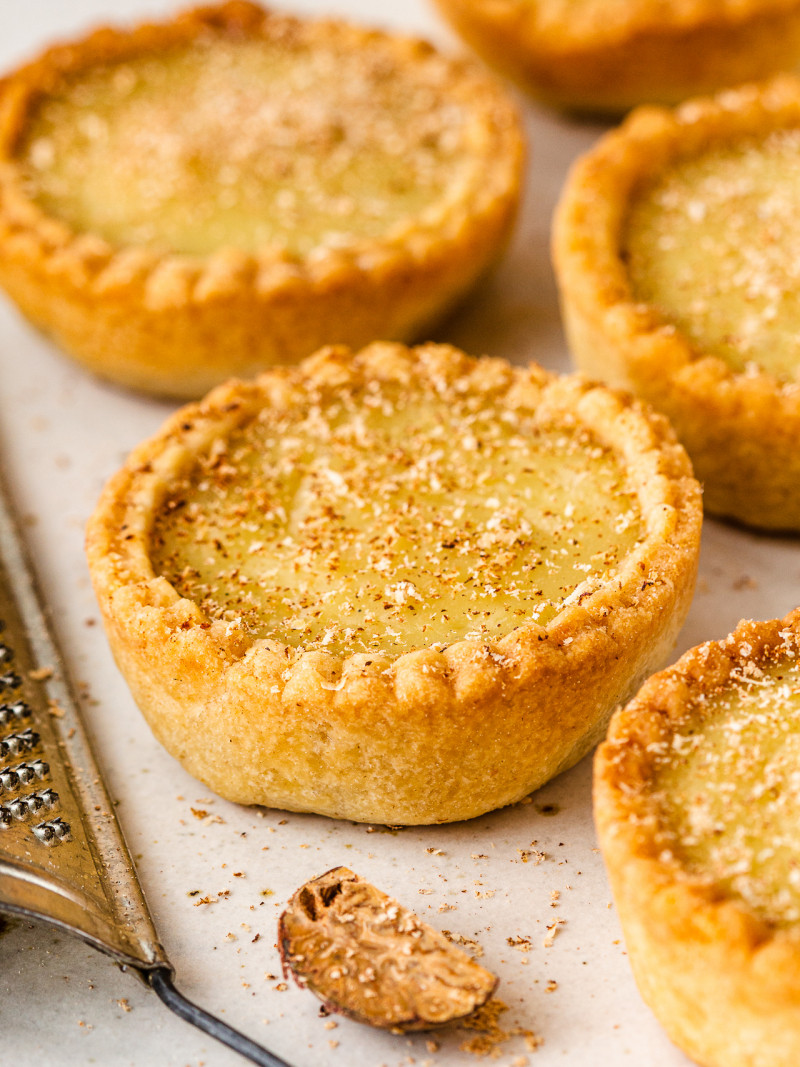This close-up food portrait captures a vibrant, indoor scene with natural light illuminating a white tabletop scattered with crumbs. Five carefully arranged, golden brown, hand-sized pies dominate the foreground, each filled with a rich lemon curd and topped with freshly grated nutmeg. To the left, an out-of-focus grater hints at the finishing touches, while a single nutmeg seed rests conspicuously on the lower right corner. In the background, additional pies, slightly blurred, frame the composition, emphasizing the delightful homemade quality of these mini tarts.